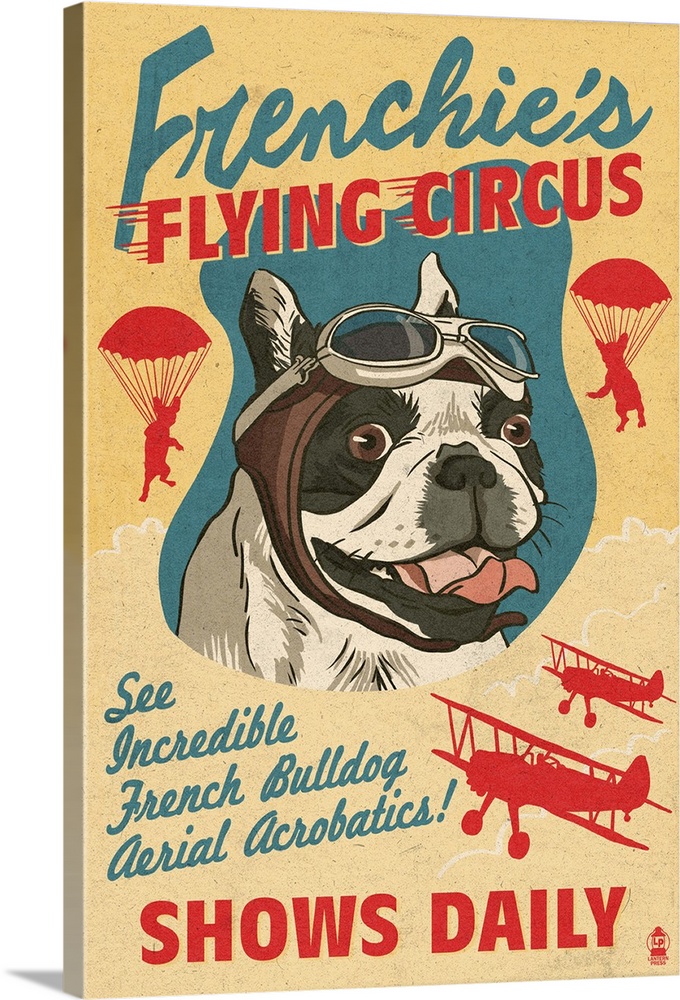The image features a decorative poster with a beige background, designed to mimic a retro advertisement for a show. At the top, in old-fashioned blue text, it says "Frenchies," with "Flying Circus" below it in bold red uppercase letters. Dominating the center is a cheerful brown and white bulldog, wearing an aviator hat with goggles resting on its forehead and its mouth open in a joyful expression. Flanking the bulldog on either side are red silhouettes of parachuting dogs. Below the central image, blue text reads, "See incredible French bulldog aerial acrobatics." To the right, two small twin-wing planes are depicted in red silhouette. The poster concludes at the bottom with the announcement, in red text, "Shows daily."